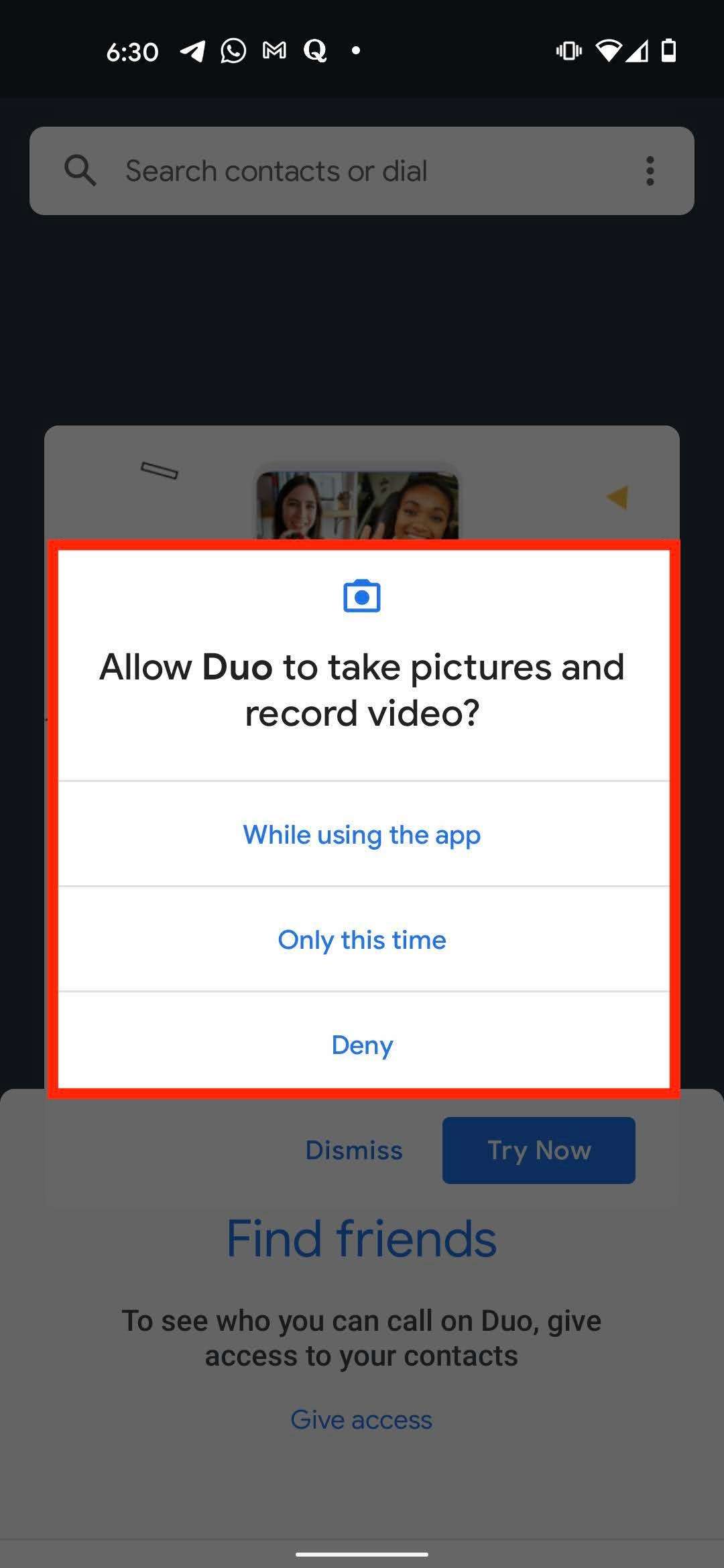The screenshot depicts a pop-up notification within a mobile phone application, partially obscuring the darkened background.

**Detailed Caption:**

The backdrop of the app is dimmed, providing a contrast that highlights the pop-up. At the top of the screen is a dark background with a prominent white search bar. Inside the search bar, a medium gray magnifying glass icon appears on the left, next to the text "Search context or dial." To the right of the search bar are three medium gray dots arranged vertically.

Below the search bar is a stretch of negative dark space, leading to a white section featuring a photograph. The photograph displays the faces of two women, positioned centrally. On the right side of this section is a yellow triangle set against a white background. To the left, at a slight angle, sits a dark gray outline of a rectangle.

In the solid background area beneath this, the word "Dismiss" is centered in blue at the top, alongside a blue button on the right labeled "Try now" in white text. Following this is the phrase "Find friends" in large blue text, centered within this part of the frame. Beneath this, in smaller black text, it states, "To see who you can call on Duo, give access to your contacts." Near the bottom, in blue text, the words "Give access" are displayed.

The pop-up in the foreground features a white background segmented by thin gray lines. At the top center of the pop-up is a blue camera icon. Directly underneath, a prompt reads, "Allow Duo to take pictures and record video," with "Duo" in bold font. There are three interaction options below: "While using the app" in blue text, "Only this time" also in blue text, and "Deny" in blue text, all aligned vertically. The entire pop-up is encased within a thick red outline.

This detailed caption comprehensively describes the image, putting emphasis on the visual elements and their arrangement for clarity.